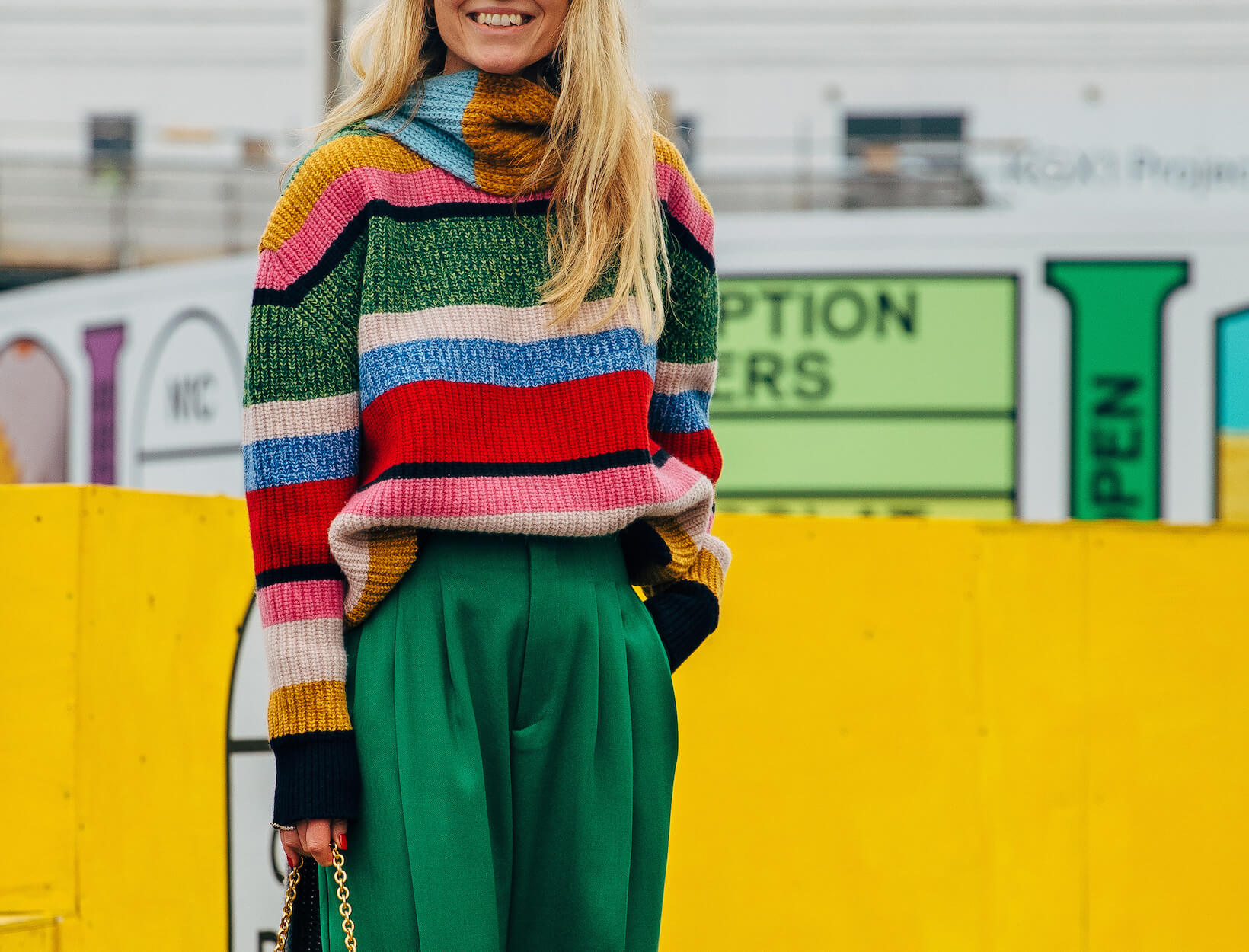The image depicts a vibrant and colorful scene featuring a blonde, Caucasian woman standing in front of a large yellow backdrop that resembles a fence. The focus is on her stylish outfit, giving the impression that this could be an advertisement for a clothing store. She is dressed in loose, pleated green trousers and a striking multicolored striped sweater showcasing horizontal bands of colors including pink, white, red, blue, green, black, and yellow. The woman is thin, and her sweater is stylishly tucked into the front of her pants. She is holding a purse, indicated by the gold chain visible near her waist, hinting at the bag being out of the frame below her thighs. The photo captures her from just below her nose down to about her thighs, highlighting her smiling face and blonde hair, complemented by a scarf around her neck. The bright background features blurred text, possibly street signs or directions, enhancing the overall vibrant and lively atmosphere of the image.